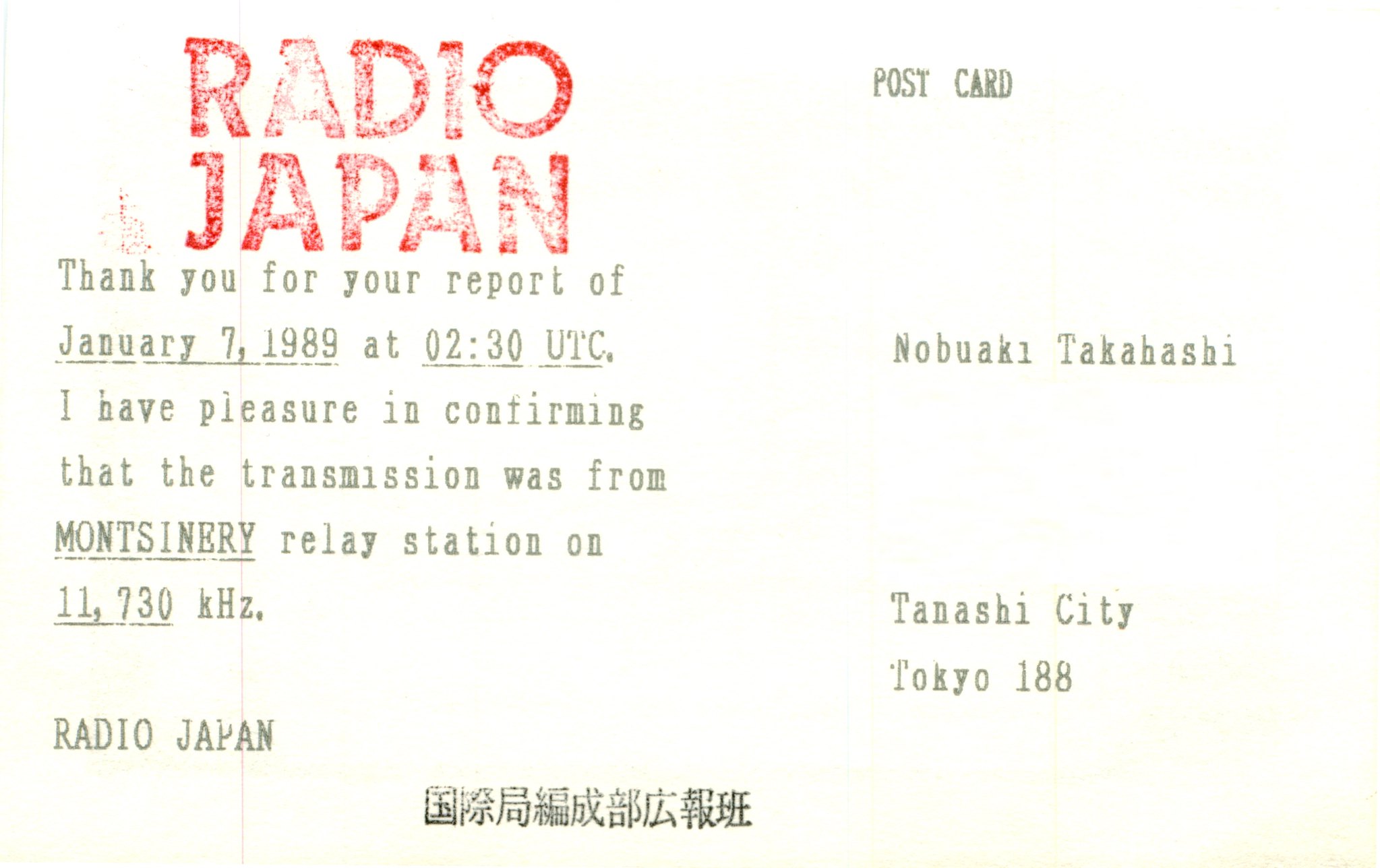This image depicts an old rectangular postcard with a light tan, slightly aged background, showing a yellowish tint around the edges, indicative of its age. In the upper left-hand corner, there is a faded red stamp that reads "Radio Japan" in bold letters. Below this, in smaller green type, the text says, "Thank you for your report of January 7th, 1989 at 0230 UTC." The date, time, and "0230 UTC" are underlined. The message continues, stating, "I have pleasure in confirming that the transmission was from Monsonary Relay Station on 11,700 KHz," with the frequency also underlined. 

In the upper right-hand corner, the word "Postcard" is typed in green. Centered in the midline of the postcard is the name "Nobuaki Takahashi," followed by "Tanashi City, Tokyo 188." At the bottom footer, within the central lower portion of the image, rows of Japanese characters are printed in black.